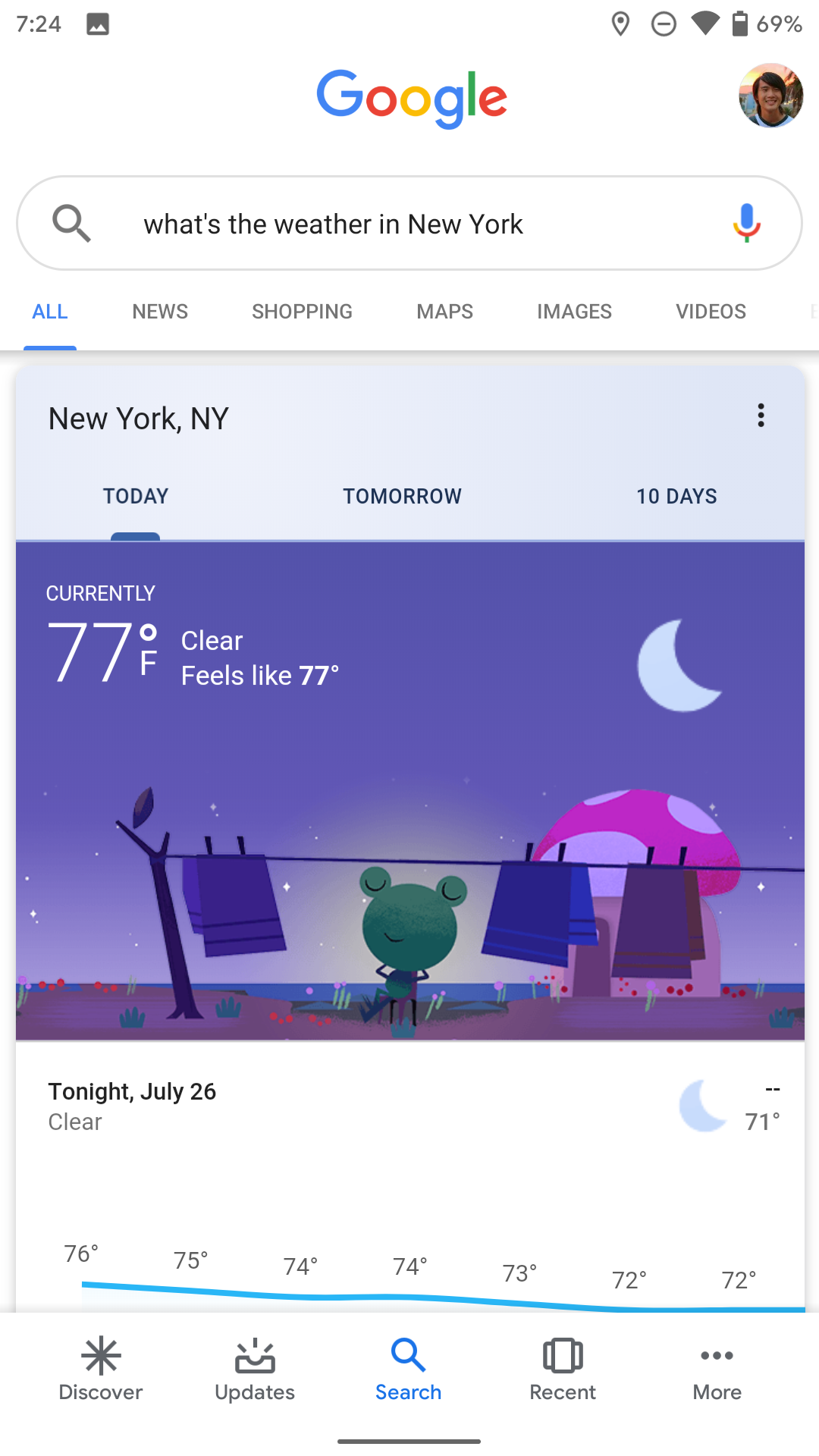This is a detailed caption for the described image:

---

The image shows a Google search result on a mobile interface. At the very top, it displays time, battery charging indicators, signal reception indicators, and a location icon, indicating that the location services are enabled. Below these indicators is the Google search bar, where the user has typed "What's the weather in New York."

Displayed prominently is a weather information card. At the top of this card, it reads "New York, NY." The card features three tabs: "Today," "Tomorrow," and "10 days," with the "Today" tab being selected.

The background of the weather card showcases an adorable cartoon illustration: a frog stands beside a whimsical mushroom house under a starry sky. A moon shines from above, and a clothesline stretches across the scene, adding a playful touch.

Overlaid on the upper left corner of the illustration is a text box that states, "Currently 77°F, Clear, Feels like 77°F." Beneath this, additional text provides further details: "Tonight, July 26, Clear," followed by a projected temperature drop from 76°F to 72°F.